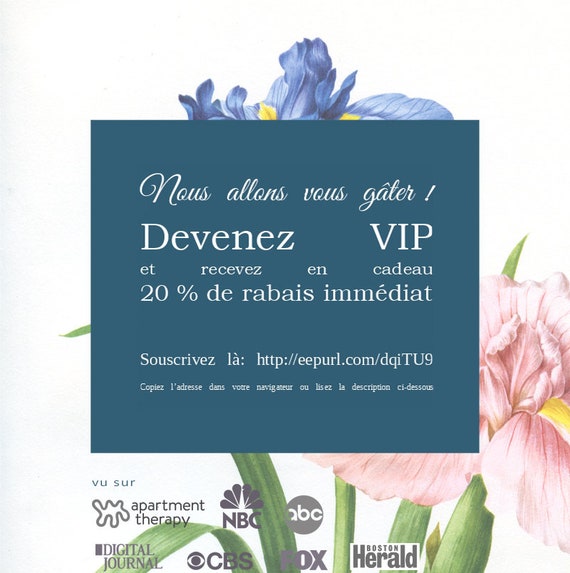This small, vertical, rectangular image appears to be an advertisement for a product, featuring a dark blue label with white French text prominently displayed in the center. The background is adorned with a beautiful floral arrangement, including lighter blue and purple irises above the label and a large pink bearded iris to the right. Stems and leaves fill in the lower portion of the background, enhancing the aesthetic appeal. 

The label's text reads: "NOUS ALLOUS VOUS GÂTER!" followed by "DEVIENEZ VIP" in bold letters, and at the bottom, "20% DE RABAIS IMMÉDIAT." The lower left corner of the image showcases various logos, including Apartment Therapy, NBC, ABC, CBS, Fox, and Digital Journal, while the right side features the Boston Herald logo.